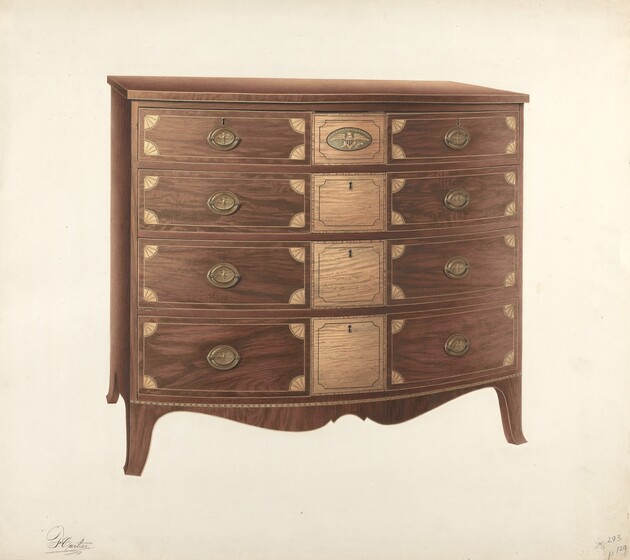This image depicts an intricately detailed brown wooden dresser, which appears to be either photographed or painted, resting on a creamy white piece of paper. The dresser exudes an antique charm, characterized by its aged appearance. It features a total of twelve drawers: eight smaller drawers adorning the left and right sides, each embellished with delicate, shell-shaped designs in the corners, and four larger drawers in the center. 

The topmost central drawer seems to have a decorative emblem, while the three drawers beneath it are equipped with keyholes, hinting that they could be locked and unlocked with a key. These central drawers are of a lighter brown hue, harmonizing with the fan-shaped adornments on the corner drawers. 

A signature that is indecipherable is located at the bottom left-hand corner of the piece, and the numbers "293P129" are penciled in the bottom right-hand corner. This meticulous depiction of the dresser offers a glimpse into a bygone era, capturing both the elegance and functionality of antique furniture.